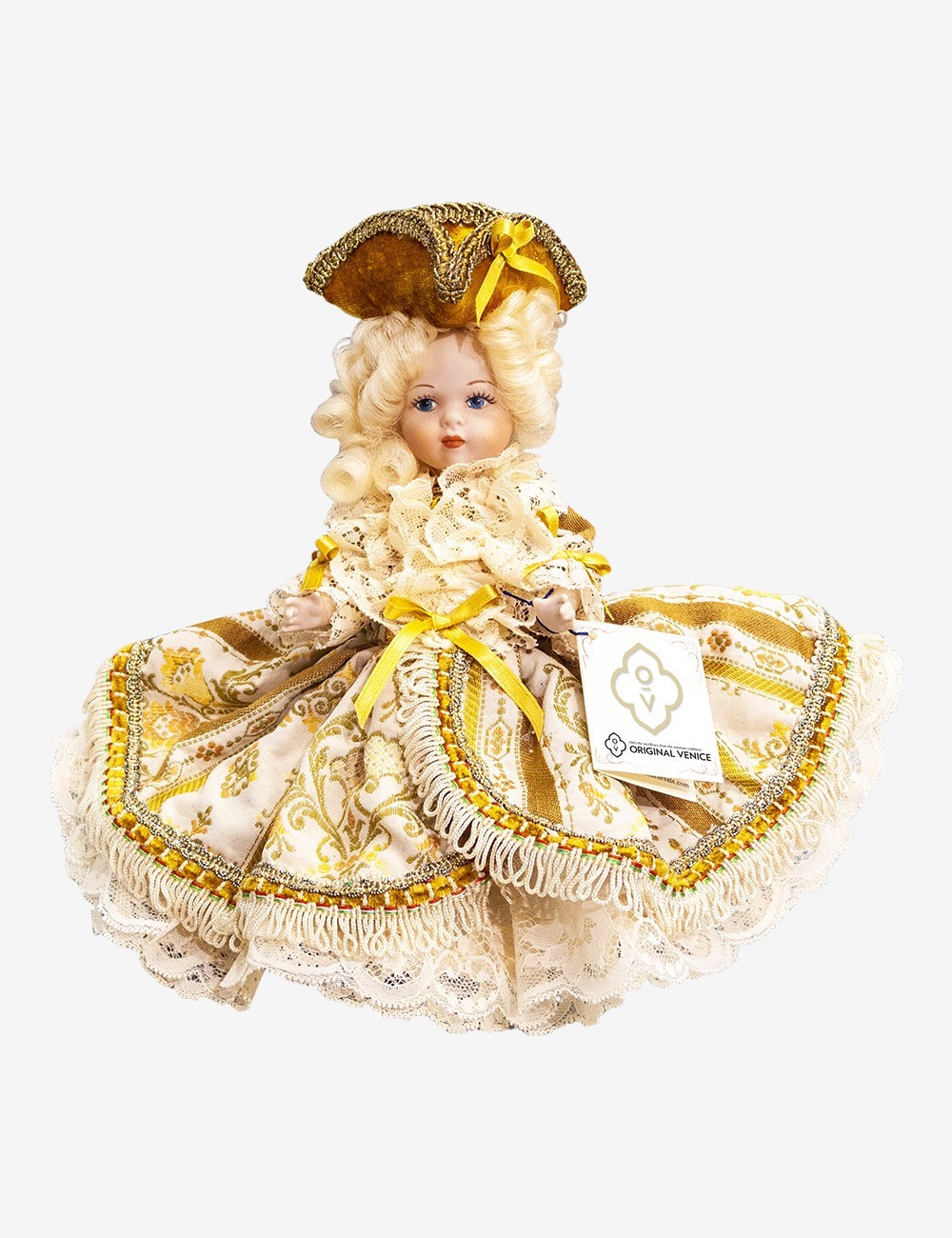This image captures a professionally photographed small doll set against a stark white background, emphasizing its intricate details. The doll features a porcelain face framed by tightly curled platinum blonde hair. Atop her head, she sports a mustard yellow hat adorned with a red ribbon accent, resembling a sailor's or pirate's hat. Her voluminous dress, filleted out elegantly, is a creamy off-white color with dark yellow and mustard yellow stripes and designs. The dress is trimmed with yellow accents and white lace, and prominently features a large yellow ribbon at the waist and a yellow border along its edges. Fleur-de-lis designs appear on the dress, adding an ornate touch. The doll's small hands are barely visible, peeking out from the sleeves that blend into the background. A tag on the side of the dress reads "Original Venice," possibly indicating the doll's origin or brand.